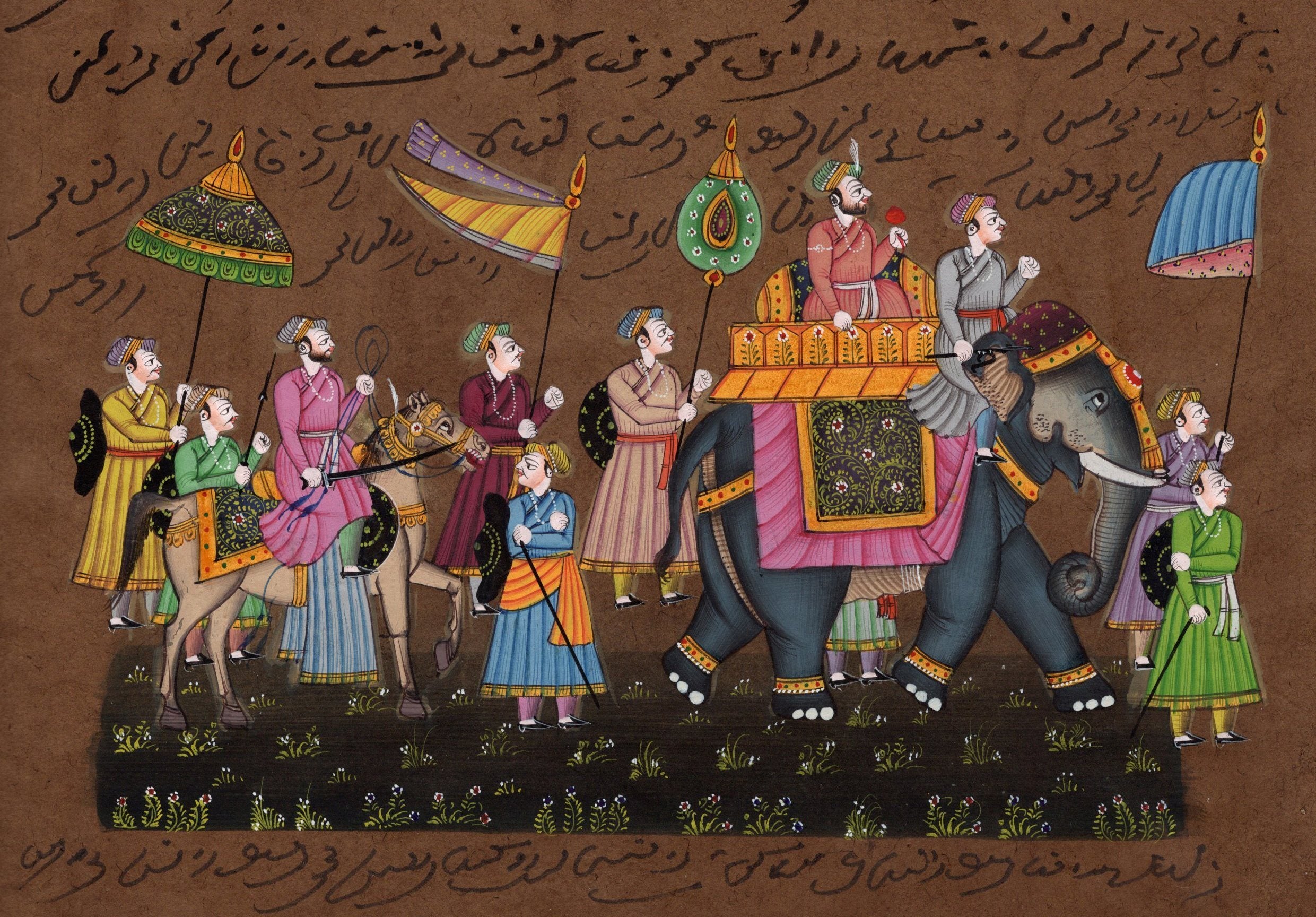This richly detailed and colorful drawing depicts a vibrant procession through a small, green, patchwork field of crops. Above and below the field are inscriptions in an unknown language, possibly Arabic, set against a brown background. At the forefront, a person in a long, flowing purple dress holds a blue and red flag, standing next to another individual dressed in green. Behind them, a magnificently adorned elephant, draped in a floral-patterned purple cloth and wearing a decorative headdress, carries two riders—one in gray and another in red. Following this majestic figure, five more individuals march, three of whom also bear flags. Among them is a man dressed in purple riding a horse. The entire scene teems with vivid colors, such as green, pink, dark pink, and auburn, reflecting traditional Middle Eastern attire. The flags and their clothing contribute to the overall vibrancy and festivity of this historical depiction.